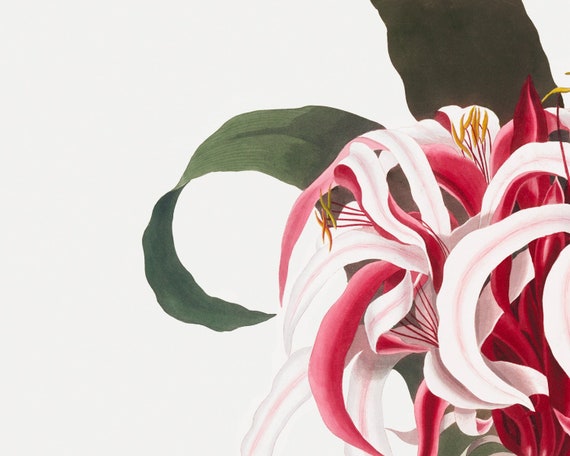This detailed illustration depicts a crinum lily, portrayed in a semi-botanical style against a stark white background. The composition is weighted towards the right half of the image, allowing the vivid colors and intricate details to stand out. The artwork features luscious, long green leaves, one pointing upward and another curling gracefully to the left. The flower, in full bloom, showcases a stunning combination of pink, red, and white petals with delicate red and pink streaks accentuating the white petals. At the heart of the flower, yellow stamens emerge, adding a vibrant contrast. The petals and leaves organically overlap, creating a sense of depth and natural fluidity in the artwork.